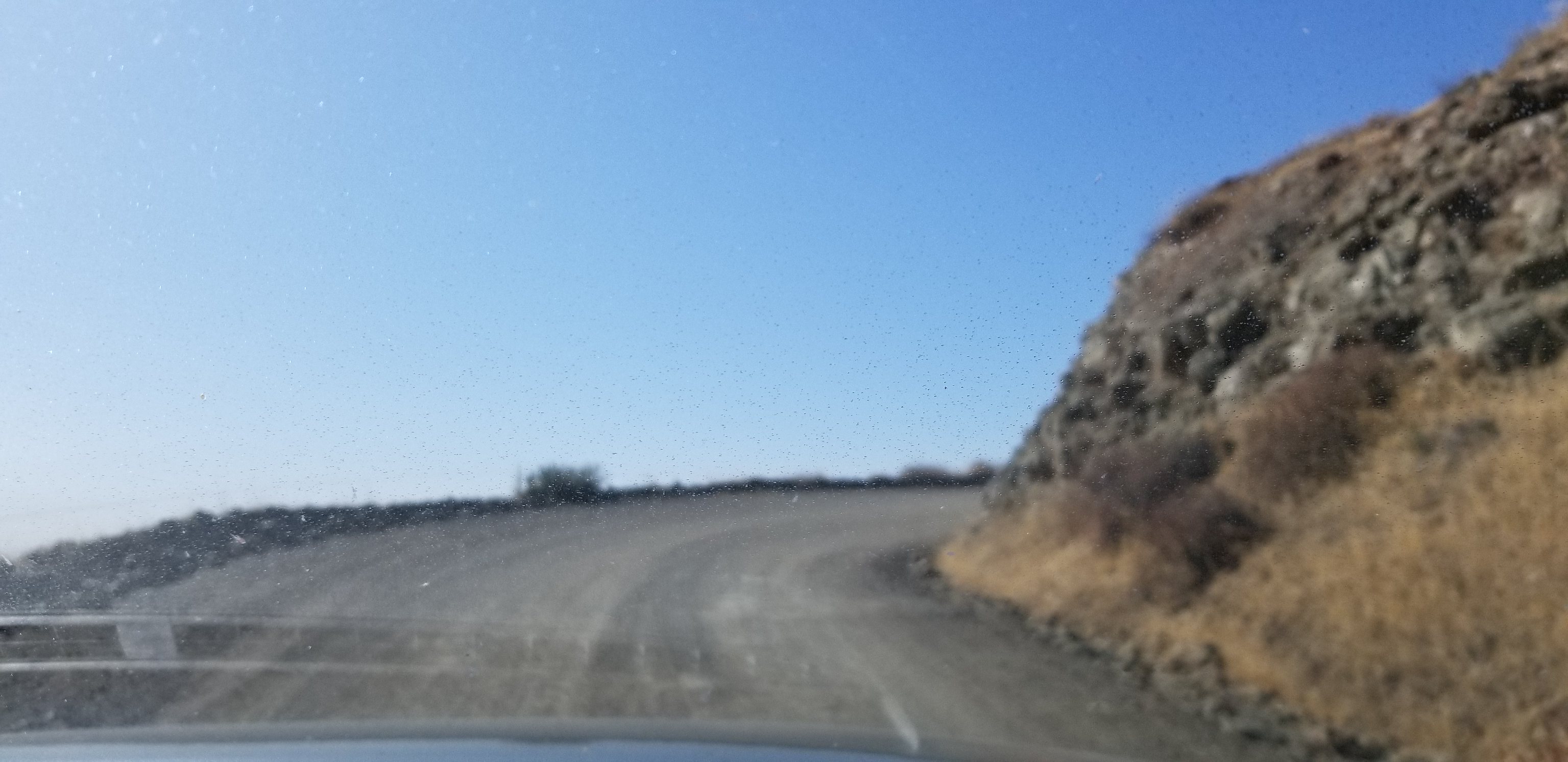The photograph appears to be taken from the passenger side of a high-clearance vehicle, likely a truck or SUV, given the elevated perspective relative to the ground. The image showcases the vehicle's right-hand side, including the hood, suggesting an off-road adventure in a desert or arid country setting. The vehicle is navigating a dirt or gravel road that may be on an incline. To the left, large rocks suggest the proximity of a cliff, although the exact nature of the drop-off remains unclear from the image. On the right, a small cliff or hill rises, supporting the idea that the terrain climbs upward in that direction. The landscape is distinctly rocky and sparse, indicative of a hot, desert climate.